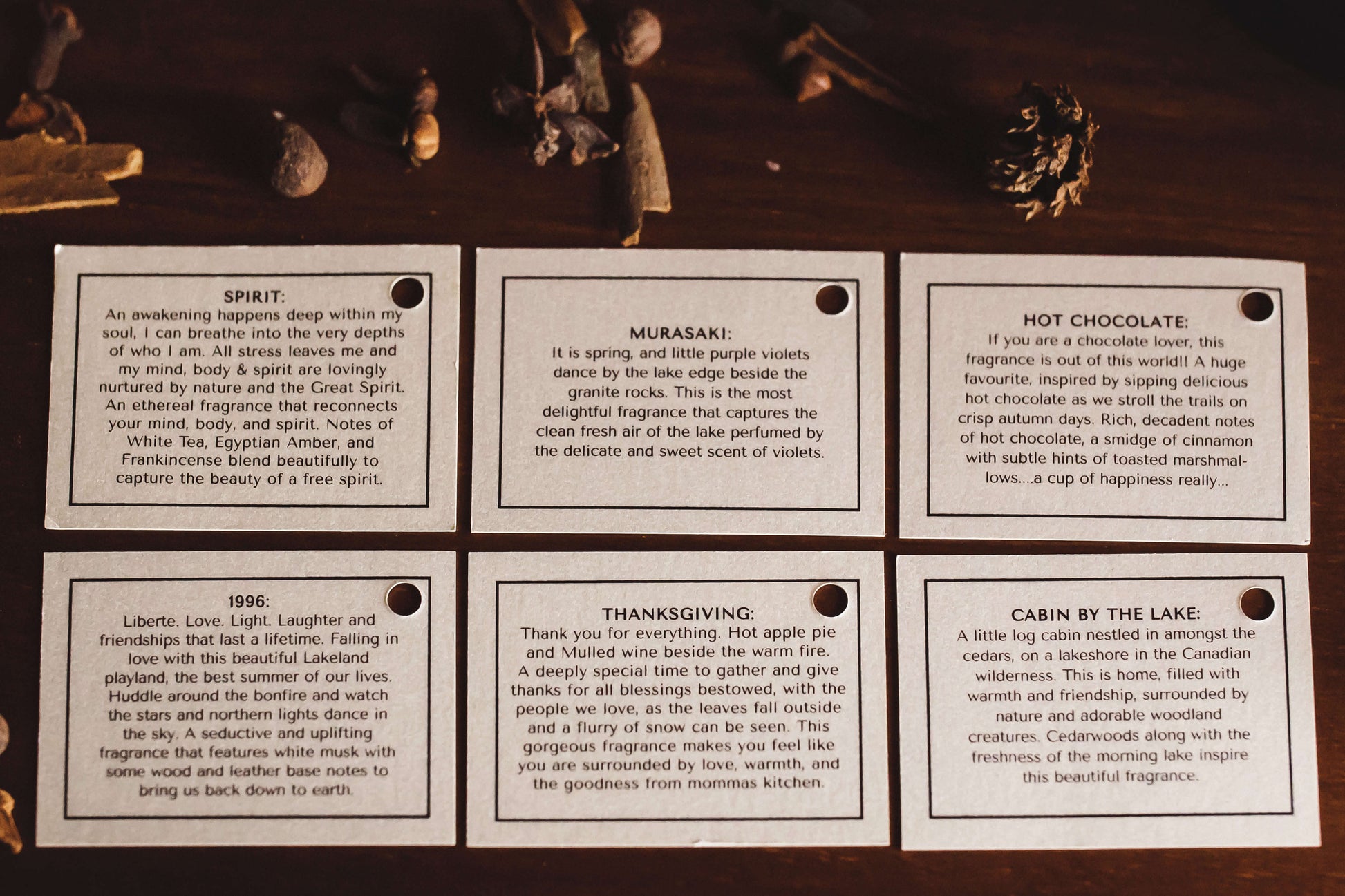The image displays six rectangular labels, each with a single bold word at the top center within a white rectangle, all laid out over a wooden table. The labels are arranged in two rows of three. From left to right on the top row, the labels read: "Spirit," "Murasaki," and "Hot Chocolate." On the bottom row, the labels are: "1996," "Thanksgiving," and "Cabin by the Lake."

Each label is bordered by a brown-outlined rectangle that has a hole on the right end, through which items can be threaded, although currently there are only a few items threaded through. The label titled "Murasaki," for example, has detailed text that reads: "It is spring and little purple violets danced by the lake edge beside the granite rocks. This is the most delightful fragrance that captures the clean, fresh air of the lake, perfumed by the delicate and sweet scent of violets." 

Above the labels, additional items such as rocks, acorns, and parts of plants are scattered on the table. The scene suggests a collection of labels with poetic texts, possibly part of a flipbook, due to the holes in each label. Despite a dimly lit setting, the arrangement and details hint at an evocative, perhaps mystical, compilation of themes.